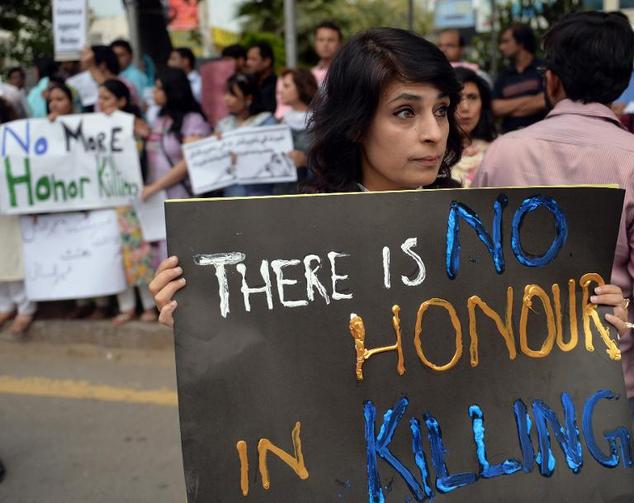This photograph captures a significant moment at a protest against honor killings. Centered prominently is a stern-looking woman with medium-length, dark brown hair, holding a black sign with the message "There is no honor in killing," written in various colors: white for "is," blue for "no," and gold for "in honor." The paper appears to be slightly peeling, indicating its likely made of black paper rather than cardboard. Behind her and extending into the background are numerous individuals, primarily women, many of whom are also holding signs expressing similar sentiments. Notably, two women to the left hold a sign saying "No more honor killing," using blue, black, and green paint. The setting appears to be a street, discernible by the visible yellow no-parking lines. Other participants, including a man in a pink jacket and another in a suit shirt, further illustrate the gathering's scale and organized nature.